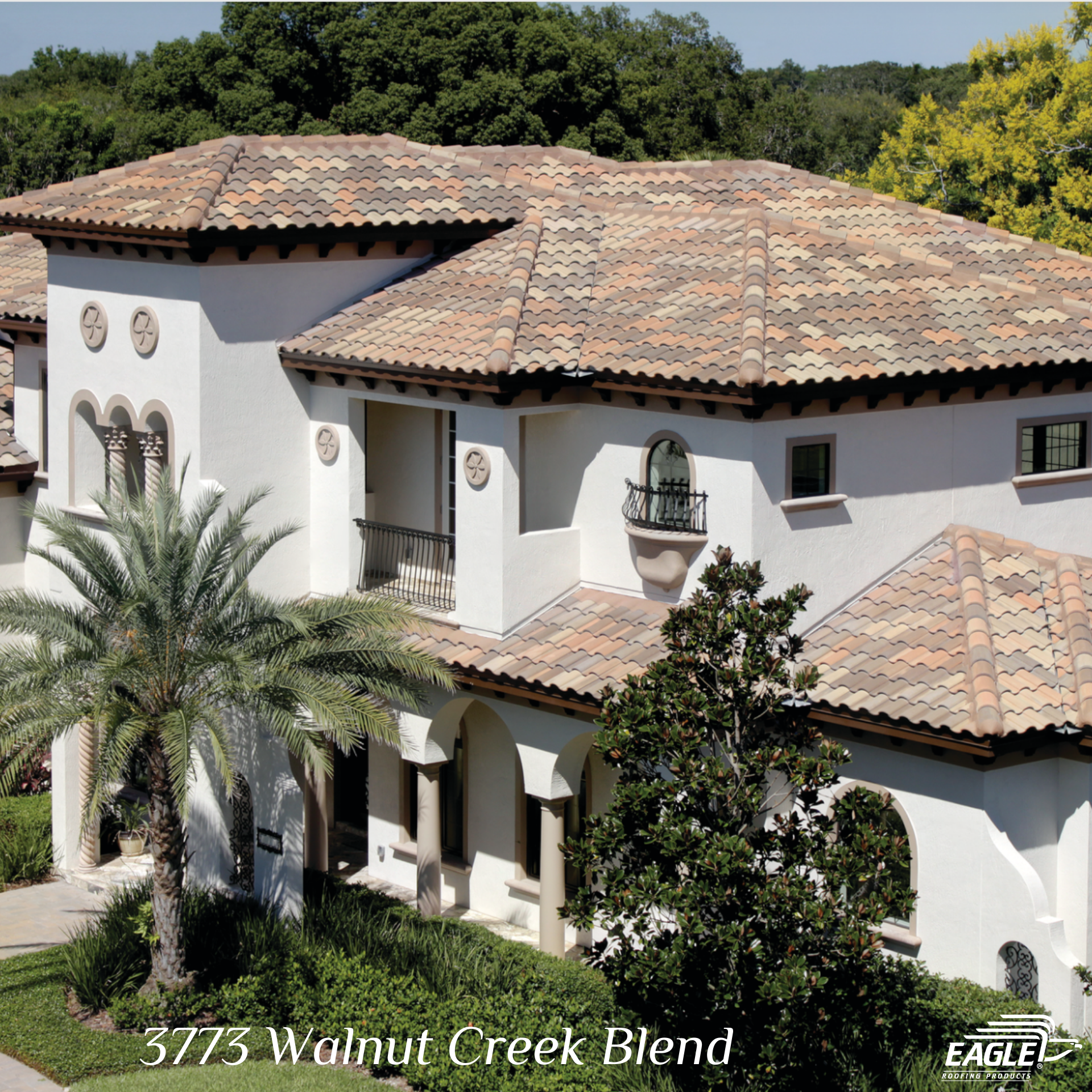The square photograph depicts an upscale, two-story Spanish-style villa, suggestive of regions like California or Arizona, adorned with a multi-colored terracotta tile roof. The roof tiles blend shades of beige, brown, terracotta, and peach, creating an intermingling mosaic of hues. The villa features white stucco walls complemented by wrought iron balconies and columns, enhancing its classic aesthetic. In the foreground, a palm tree and another tree are planted amidst a landscaped front yard, while the background reveals an expansive wooded area with treetops extending into the distance. Overlaid in white text at the bottom left is the address "3773 Walnut Creek Glen," and on the bottom right is the "Eagle Roofing" logo, depicting the outline of an eagle. This image is likely part of an advertisement for the roofing tiles themselves.